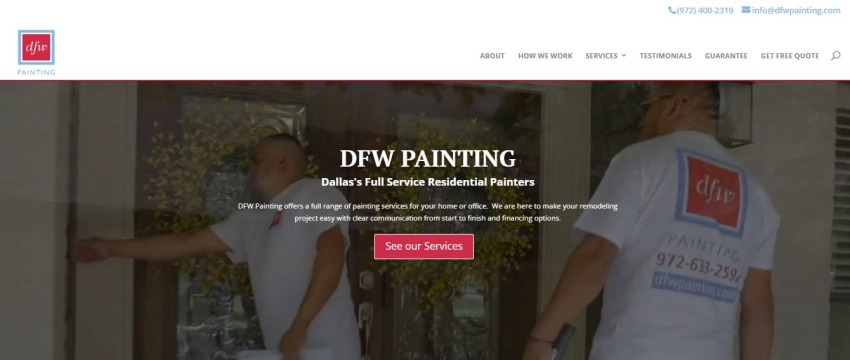This image is a screenshot of a website, which appears small and difficult to read. In the top right corner, there is a blue phone number and an email address for the company. This information is situated within a white bar that runs across the top of the page. 

On the left side of the white bar, there is a blue square outline containing a red block with the letters "DFW" inside it—D for Donald, F for Freddie, and W for Work. Below this block is the word "Painting" written in blue.

To the right of this logo, the white header bar includes navigation options: "About," "How We Work," "Services" with a drop-down menu, "Testimonials," "Guarantee," and "Get a Quote," followed by a search icon.

Below the header bar, there is a photograph overlaid with an opaque dark layer. The image depicts two men, each wearing white t-shirts, arriving and ringing a doorbell. The men have the same logo on the front left side of their t-shirts, and a larger version of the logo with the phone number and website address is printed on the back.

In the center of this photograph, on the dark overlay, "DFW Painting, Dallas's Full-Service Residential Painters" is written in white text. Below this, there are two lines of very small text, followed by the call-to-action "See Our Services," which is in white text on a red block.